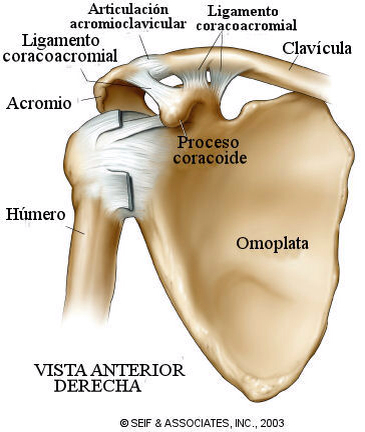The image is a detailed, computer-generated anatomical diagram from a textbook, showcasing the right shoulder joint and its components. The diagram is predominantly labeled in Spanish, providing a comprehensive view of the bones, ligaments, and tissues involved. Key elements identified include the clavicle (Clavicula), the acromion (Acromio), the humerus (Humerio), and the scapula (Omoplata). The bone structures are depicted in a light brown color, while the ligaments and connective tissues are illustrated in white. Notable annotations include "Ligamento Coracoacromial" and "Articulación Acromioclavicular." The bottom of the image features the caption "Vista Anterior Derecha," indicating this is an anterior view of the right shoulder. Additionally, there is a small reference to "CF & Associates, Inc., 2003," suggesting the image's origin or publication information.